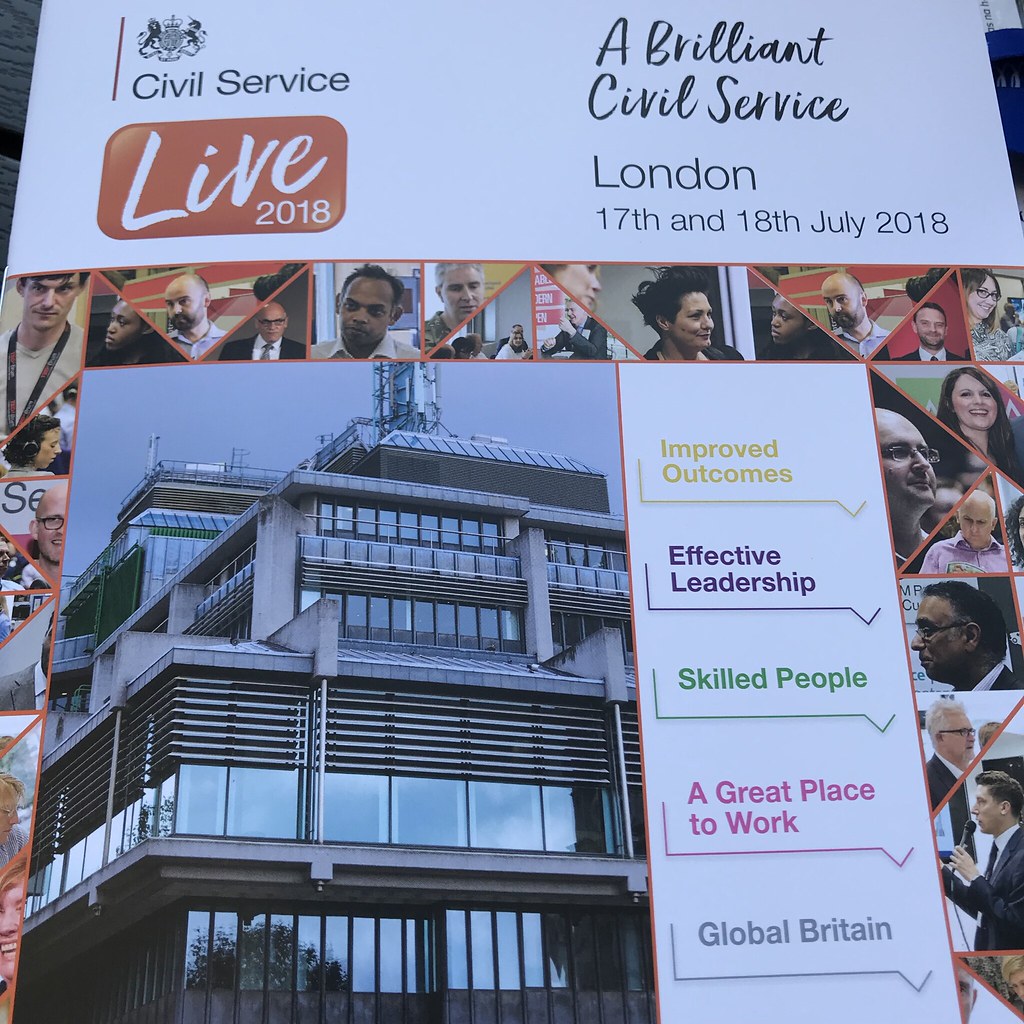The billboard advertisement is a long vertical wall scroll featuring several detailed elements. At the top, on a white background, black text reads "A Brilliant Civil Service," followed by "London 17th and 18th July 2018" in the top right corner. In the top left corner is a small logo of two lions holding a gauntlet, beneath which "Civil Service" is written. Adjacent to this, in a red rectangular bubble, white text reads "Live 2018."

Below this header is a colorful collage of mainly facial pictures forming a border. The center of the billboard showcases an image of a multi-storied office building, approximately four stories tall. To the right of this central image, between the collage and the building picture, a series of words in different colors are displayed: "Improve Outcomes" in yellow, "Effective Leadership" in purple, "Skilled People" in green, "A Great Place to Work" in pink, and "Global Britain" in blue. The overall design emphasizes a professional and vibrant atmosphere, aligning with the theme of a civil service event.